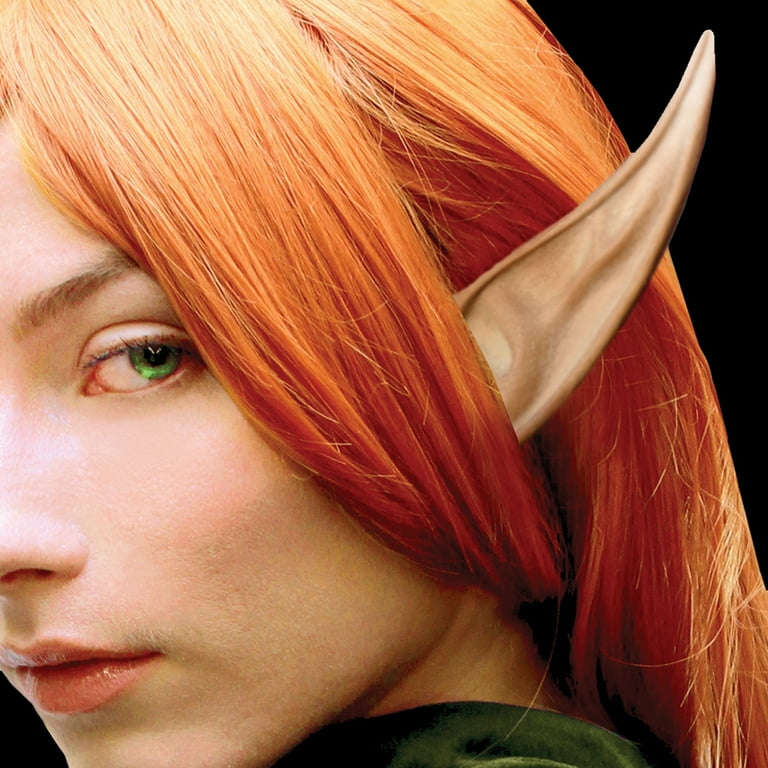The image features the close-up side view of a Caucasian girl with vibrant orange-red hair and striking green eyes. Her eyebrows are a brownish color, and her lips are a reddish hue. Notably, she is wearing a flesh-colored, slightly grayish pointed ear accessory, which makes her resemble an elf, possibly as part of a Halloween costume. Her hair, which has a somewhat plastic-like appearance, twines in front of and behind the pointed ear. She is dressed in a dark green top, visible beneath her hair. The background of the photo is all black, making her head the focal point of the image. Only one eye and one side of her face are visible, as the rest is cut off by the frame.